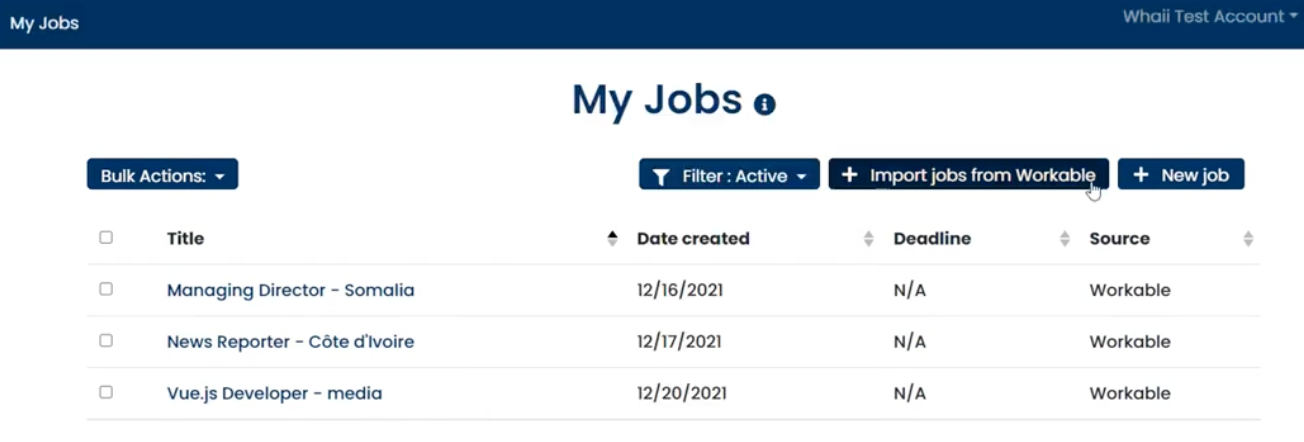The image is a small, rectangular screenshot of a likely website or app interface, focusing on job management functions. In the upper left corner, the title "My Jobs" is prominently displayed in white text against a blue, rectangular background. Directly underneath this is the same "My Jobs" title, written in dark blue text on a white background. 

On the left side, there is a dark blue, rectangular button labeled "Bulk Actions" in white text, which produces a drop-down menu when clicked. Below this button is a vertical list of checkboxes aligned one above the other. Next to these checkboxes, column headings indicate different categories: "Title," "Date Created," "Deadline," and "Source," running horizontally across the image.

Above these headings are three buttons, each producing a drop-down menu. The first button has a dark blue background, white text that reads "Filter: Active," and is rectangular in shape. The second button, slightly longer, features an even darker blue background, white text reading "Import Jobs Remarkable" with a plus sign, and it too is rectangular. The third button, with a medium blue background and white text stating "New Job" alongside a plus sign, is shorter than the second button but still rectangular.

Overall, the interface elements are neatly arranged, with clear categorizations and functionalities for managing job-related tasks.